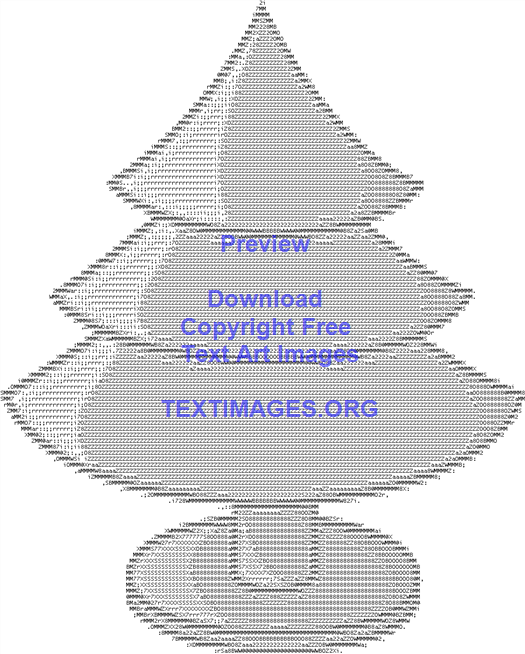This black-and-white image depicts a vertically oriented, text-based representation of a Christmas tree. The tree is meticulously crafted using ASCII text characters, with darker text simulating shadows and lighter text representing illuminated areas. The tree design includes three distinct tiers, a narrow trunk, and a broad, rounded base. Superimposed in blue text across the middle of the tree are the words: "Preview, download copyright-free text art images." Below this, it reads "textimages.org." This striking text art advertises a repository for free text-based images available for download from the mentioned website.